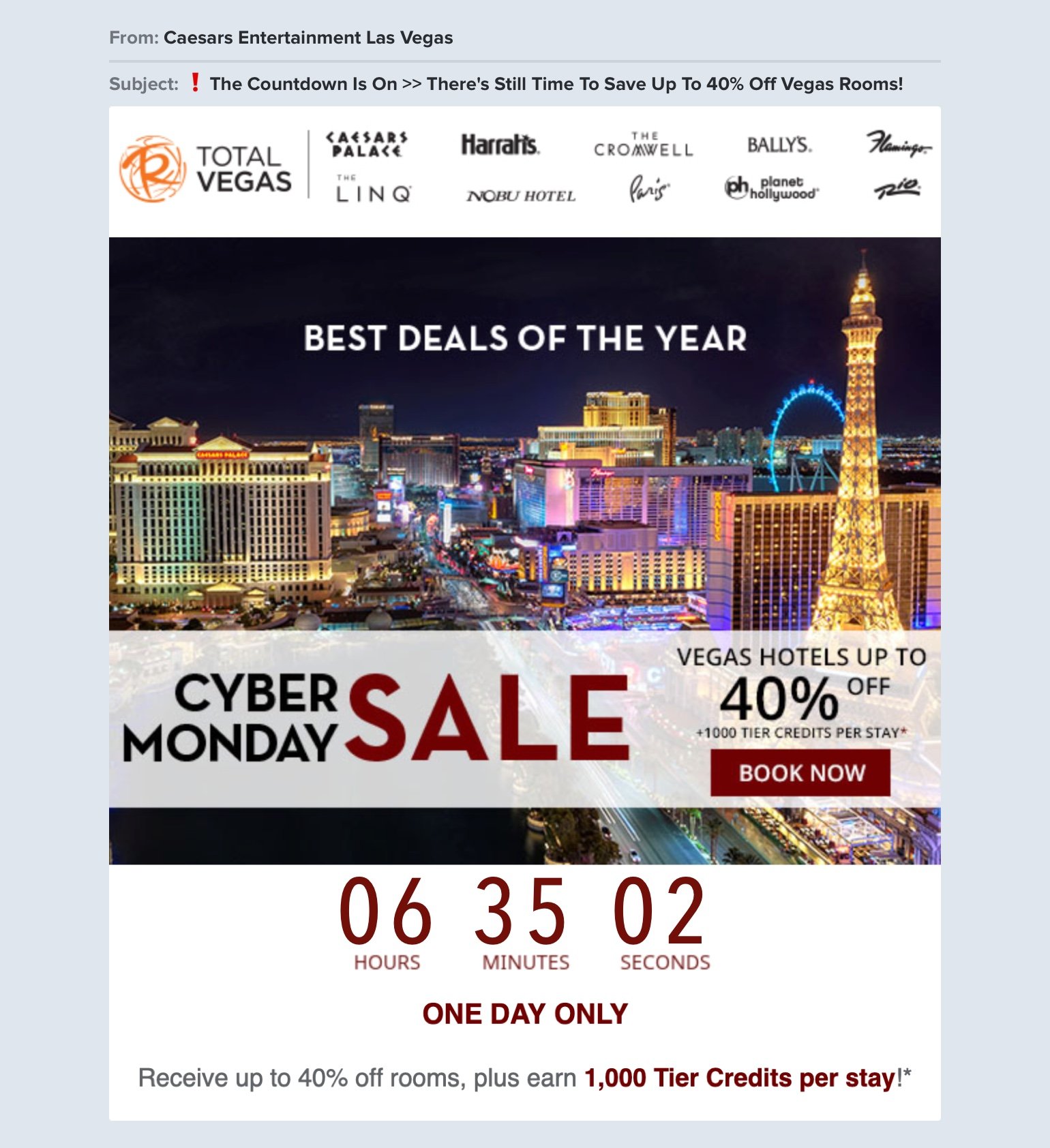**Promotional Email from Caesars Entertainment Las Vegas: Cyber Monday Sale**

**Image Description:**

The email showcases a promotional campaign from Caesars Entertainment Las Vegas, highlighting a Cyber Monday sale. The offer promises savings of up to 40% on Las Vegas hotel rooms.

At the top of the email, there’s a bold headline in white text declaring "Best Deals of the Year" followed by an even larger text that reads "Cyber Monday" and "Vegas Hotels Up to 40% Off". A prominent "Book Now" button is situated below these texts.

Key details include:
- **Logos** of several Las Vegas hotels and casinos part of the Caesars Entertainment portfolio are prominently displayed. These include Caesars Palace, Harrah’s, The Cromwell, Bally’s, Flamingo, The LINQ, Nobu Hotel, Paris, Planet Hollywood, and Rio.
- A **nighttime image of the iconic Las Vegas Strip** serves as the background, featuring brightly lit landmarks such as the replica of the Eiffel Tower, The LINQ Ferris wheel, Treasure Island, and the Bellagio.

A **countdown timer** on the email shows exactly "6 hours 35 minutes and 2 seconds" left, emphasizing the urgency of the sale. Right below the timer, text in bold red reads "One Day Only," urging immediate action. Additionally, the email mentions that customers can earn 1,000 tier credits on the first day of booking.

Overall, the layout is clean and visually appealing, designed to motivate viewers to take quick advantage of this limited-time offer and plan their next adventure to Las Vegas.